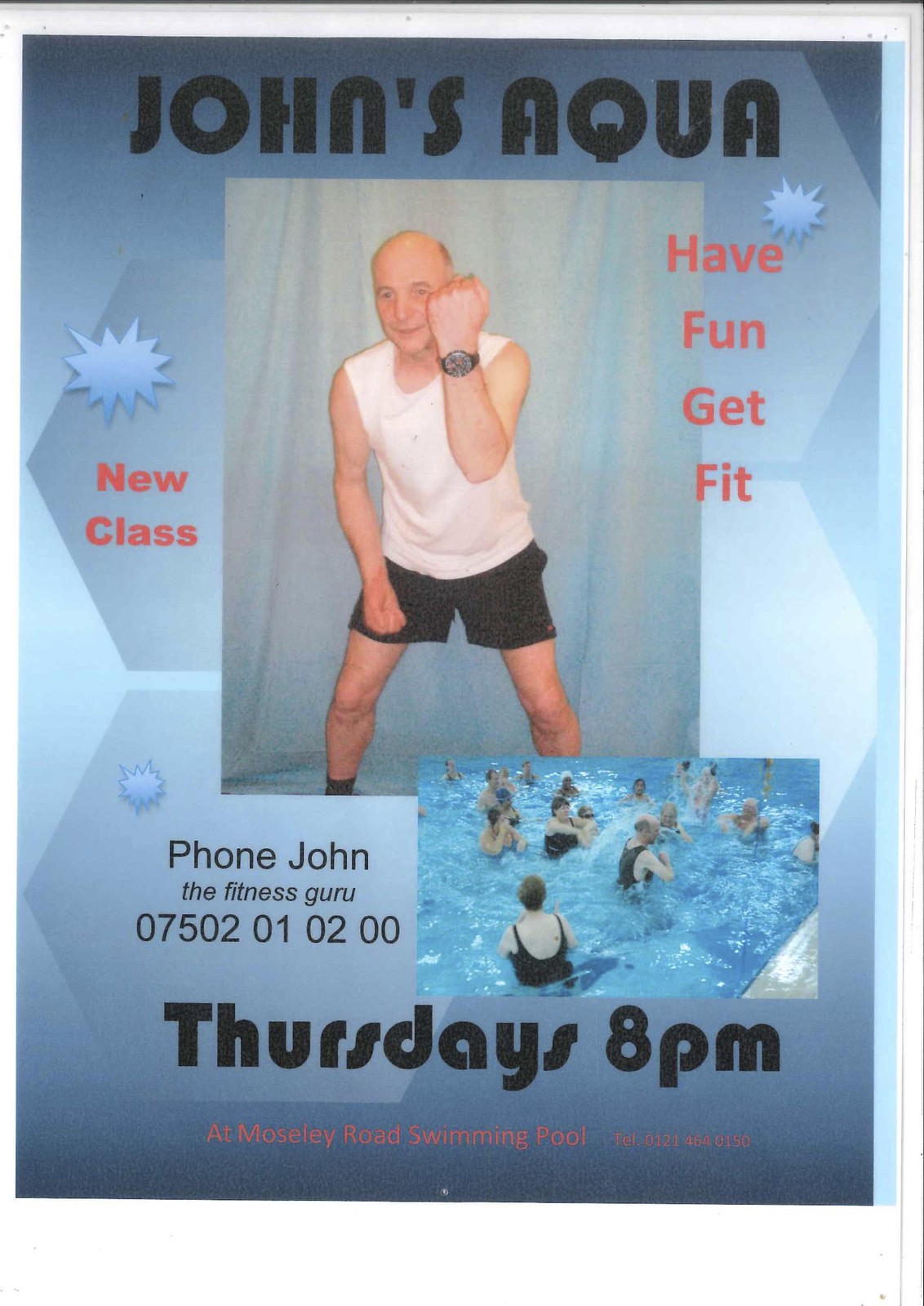The promotional flyer for a fitness event features a striking blue background with darker blue hexagon patterns. At the top, bold black text announces "John's Aqua." Dominating the center of the poster is a large photograph of a bald man in black shorts and a sleeveless white shirt, posed with his fist raised and sporting a black wristwatch. Flanking this image, red text reads "New Class" on the left and "Have Fun, Get Fit" on the right. 

Beneath the photo, black text provides contact information: "Phone John the Fitness Guru 07502010200." Adjacent to this, a small inset photo shows several individuals, likely senior citizens, engaging in activities in a waist-high swimming pool. The schedule is prominently displayed in black text at the bottom, indicating "Thursday's 8pm," with additional red text specifying the location: "At Moseley Road Swimming Pool."